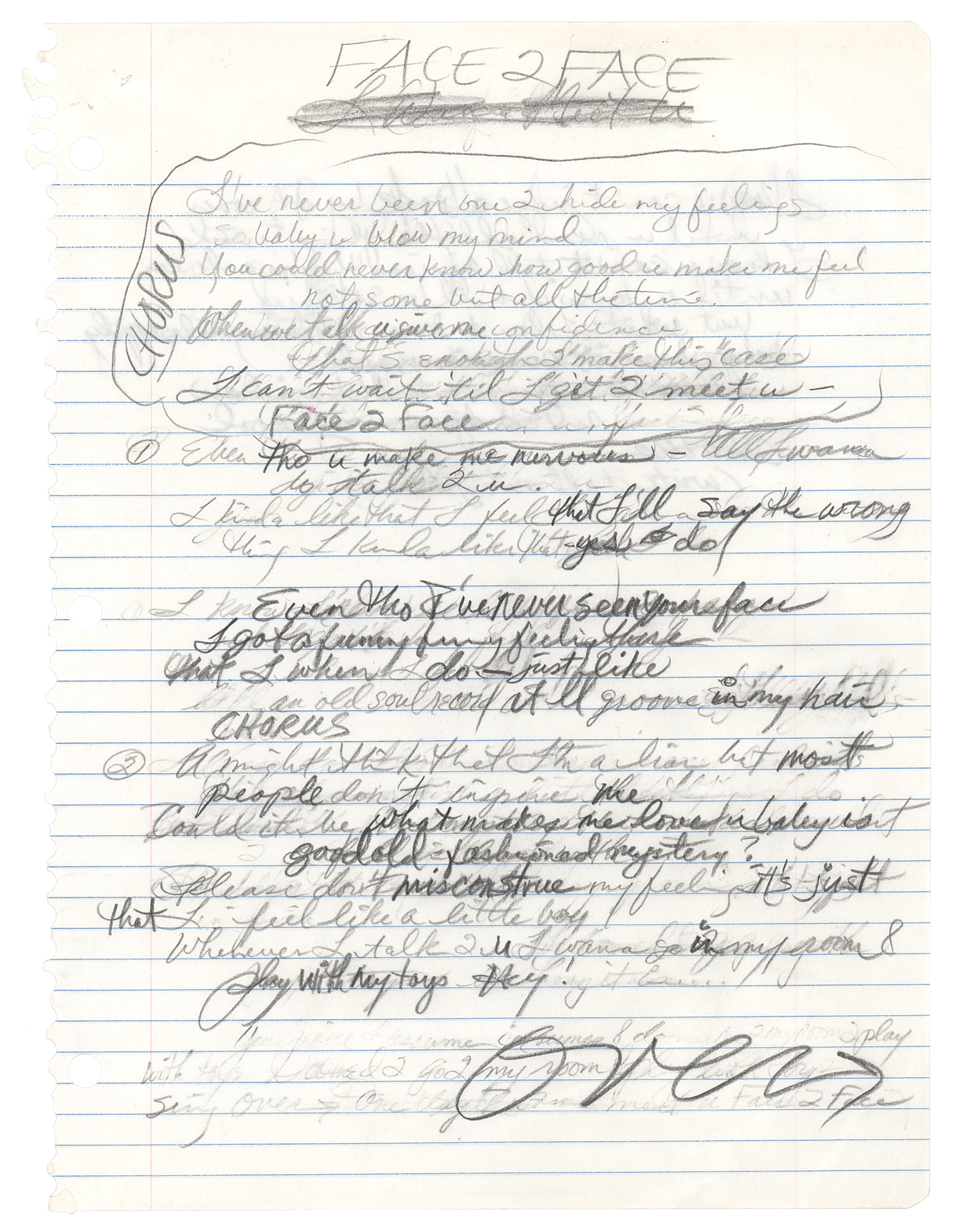This vertical image captures a handwritten rough draft of a song titled "Face to Face" on white, loose-leaf, three-hole punched notebook paper, characterized by horizontal blue lines and a vertical red margin line. The entire page is filled with messy, rushed pencil writing, indicative of a work-in-progress. The song's chorus is marked and appears multiple times, stating: "I've never been one to hide my feelings, baby, blow my mind. You could never know how good you make me feel." Additional decipherable lyrics include lines about gaining confidence while talking and feeling a special connection despite never having met face-to-face. The handwriting varies in darkness, suggesting some lines were traced over for emphasis. An arrow at the bottom of the page indicates there is more to the song on the following page.